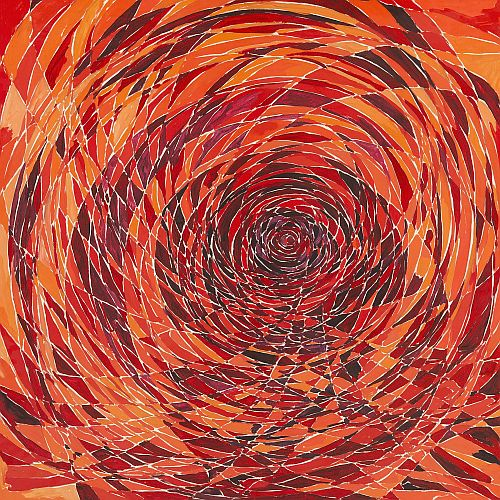This is an abstract painting depicting a swirling vortex that converges at the center, creating the illusion of looking down a tunnel. The vortex is formed by rounded, thin white lines that draw the eye inward, enhancing the tunnel-like appearance. The walls of the vortex are vibrantly colored in various shades of orange and red, starting from light yellowish-orange at the outer edges and intensifying into deep reds, burgundies, and purples as they approach the center, which is a dark, almost black burgundy. The swirling pattern is intricately detailed, interspersed with triangular forms and quadrilaterals in red, green, and brown hues. These shapes are connected by white lines that contribute to the abstract, kaleidoscopic effect, and they become increasingly elongated nearer to the center, forming a rough circular pattern. Though the painting uses a unified color scheme to convey a sense of harmony and simplicity, closer inspection reveals a rich, textured interplay of shapes and shades. There is no signature visible on the painting, and the overall composition emphasizes a perspective that draws the viewer into the central point, evoking a tangible sense of depth and motion.